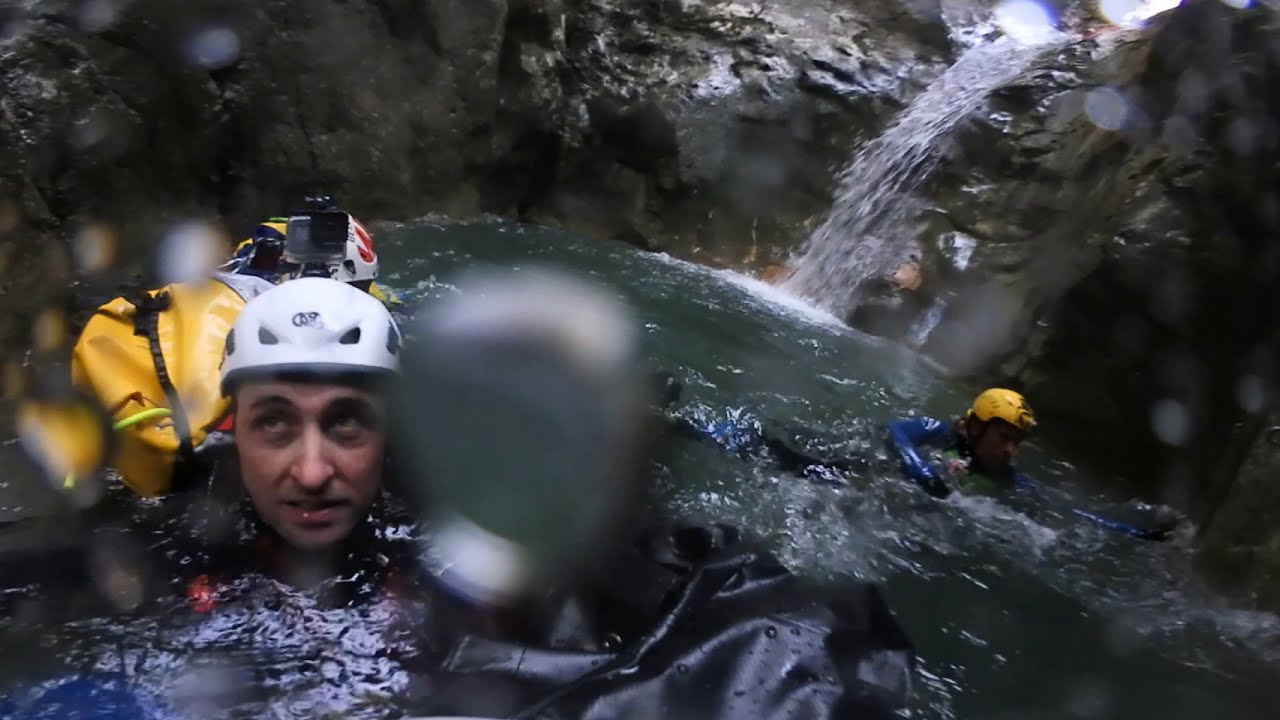In this detailed image, a small body of water occupies the center, with a waterfall cascading down into it from the top right, creating a serene yet dynamic focal point. The scene is illuminated by natural daylight, revealing a setting that appears to be deep within a cave system, surrounded by wet and shiny rocks. Two individuals, both submerged up to their waists in the water, are engaged in exploration. The individual closest to the camera is wearing a white helmet and has a yellow backpack floating nearby. Another person, positioned slightly to the right and further back, sports a yellow hard hat and is equipped with blue swim gear. Both are spelunkers or cave explorers, underscoring the adventurous atmosphere of the image. The lens displays a few water droplets, adding to the sense of immersion. The overall palette includes shades of green from the surrounding moss and flora, accented by the explorers' bright equipment, in hues of white, yellow, red, and blue.